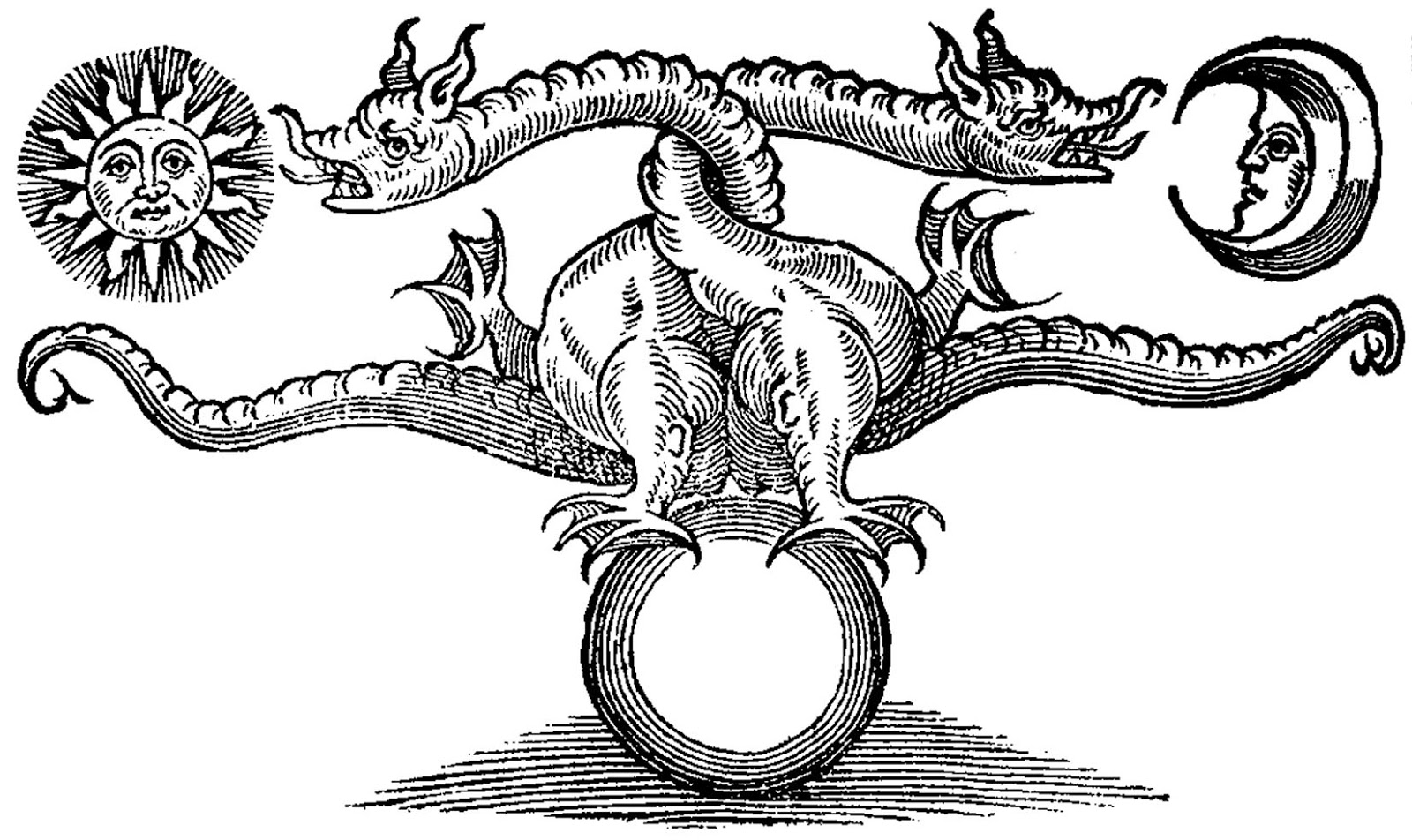A detailed black-and-white sketch is presented against a white background, devoid of any border or text. In the upper left corner of the image, a solemn-looking sun with a face, complete with eyes, nose, and mouth, radiates rays in all directions. On the right side, a crescent moon with a neutral expression is depicted, featuring a face within its curved interior. At the image's center, toward the bottom, a circular wheel-like object stands upright, characterized by a white center. Perched on this wheel are two intertwined dragons with open mouths that give them an angry appearance. The dragon on the right, twisted to face the left, directs its gaze at the sun. Conversely, the dragon on the left, twisted around the former, faces the crescent moon on the right. Their bodies and legs are detailed with curled tails stretching horizontally beneath them, adding an intricate layer of symmetry to the composition.